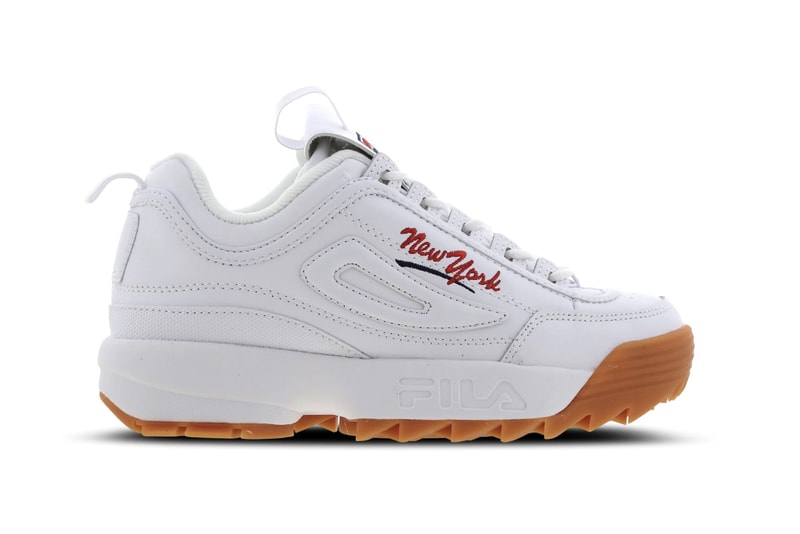The photograph features a single, white Fila sneaker that appears to be staged against a pure white background. The sneaker sports white laces and a prominent red and black label on the side, with "New York" elegantly written in red cursive, accompanied by a black swooping line beneath it. The toe and bottom sections of the shoe are made of a light brown rubber material, designed to offer a good grip with its ridged sole. Additionally, there is a convenient white tab at the back of the shoe, presumably to aid in sliding it on. While the sneaker looks robust, its actual weight is uncertain. The overall minimalist presentation draws focus solely to the detailed features of this Fila sneaker.